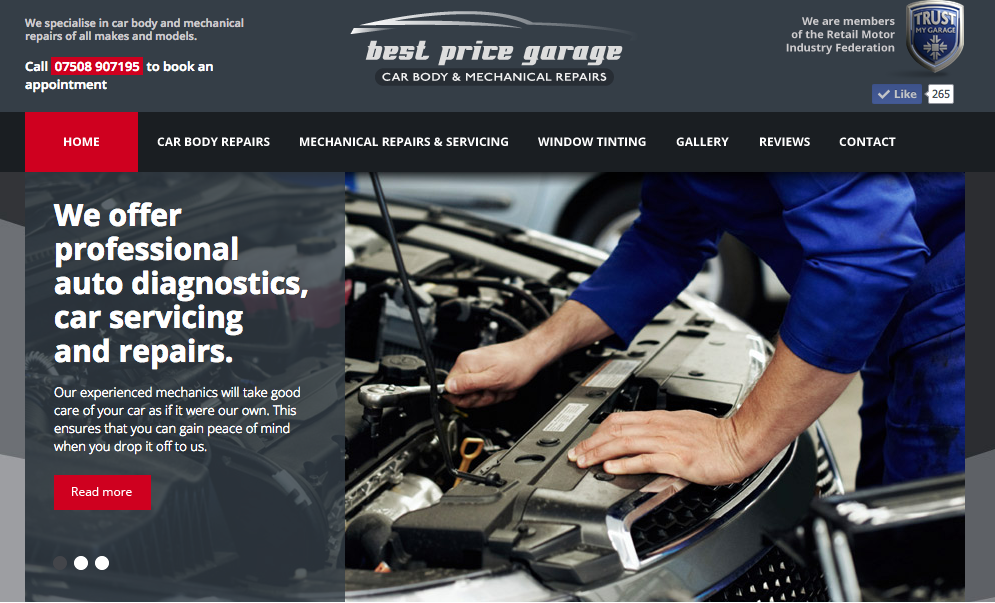The image depicts a highly detailed webpage for an automotive repair business. The background at the top is gray with prominent white text. On the top left corner, there is a red-highlighted text stating "Call 07508-907-195 to book an appointment." Centrally positioned at the top is the business name, "Best Price Garage, Car and Body Mechanics Repair." On the right side of this header, it mentions membership with the "Retail Motor Industries Federation" followed by a blue and gray shield that has the word "Trust" on it. Directly below this shield, a button shows a like count of 265.

The left side of the page is demarcated by a red-highlighted 'Home' button, followed horizontally by navigation links titled "Car Bodies," "Mechanic Repairs and Servicing," "Window Tinting," "Gallery," "Reviews," and "Contact."

Centered at the bottom of the image is a photograph of a car with its hood open. A man dressed in blue overalls is working on the car, holding a ratchet. To the left of this image, a text block reads, "We offer professional auto diagnostics, car servicing, and repairs. For experienced mechanics, we'll take good care of your car as it were. This ensures that you gain peace of mind when you drop it off to us." Below this text, a prominent red button with the text "Read More" invites further engagement.